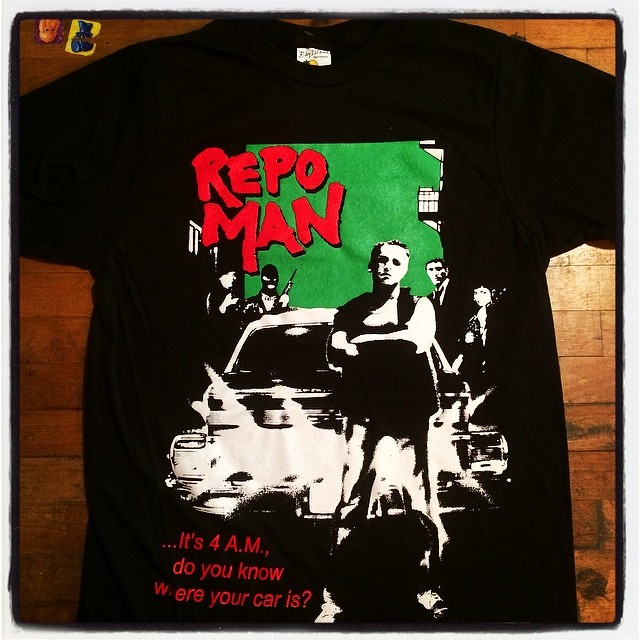The image features a black t-shirt spread out on a wooden background with a medium brown hue. The shirt prominently displays a bold, detailed design. At the top of the shirt, the words "Repo Man" appear in red graffiti-like font within a green square. The main graphic showcases a man with a defiant posture, arms crossed, standing in front of a car. He has his head slightly tilted, exuding an assertive attitude. Behind him, multiple figures, including a masked man holding a firearm, are depicted in silhouette. Additional background details include the awning of a building and some stairs in the top left corner. At the bottom left of the shirt, red text reads, "It's 4 a.m. Do you know where your car is?" The shirt is laid out in a manner that fully displays the entire graphic, including the small size and visible inside collar tag.